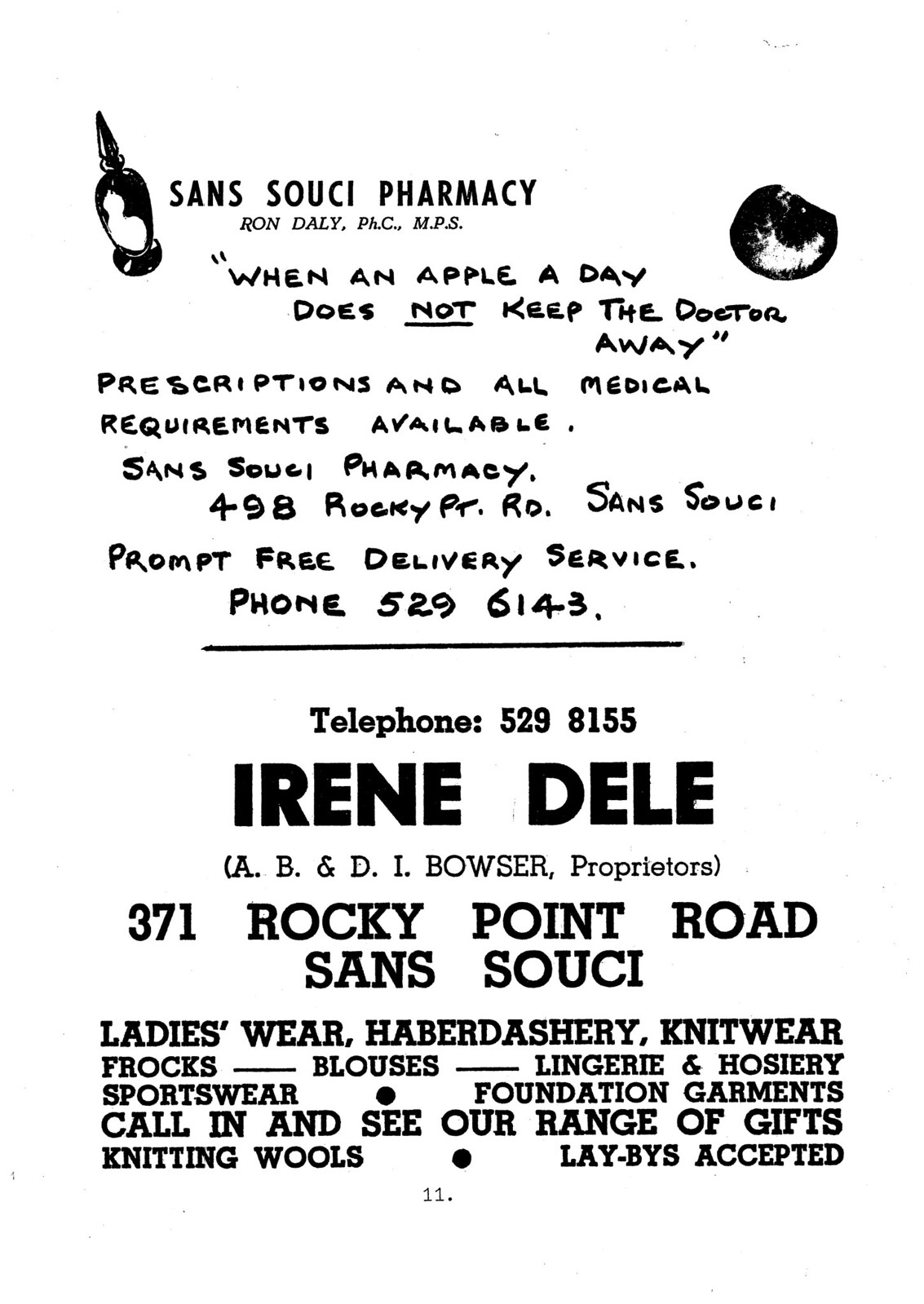The black-and-white print advertisement, appearing on page 11 in portrait orientation, is divided into two distinct sections. The top half features an ad for Sans Souci Pharmacy. To the left, there's a line art depiction of a pharmaceutical bottle, and to the right, a pen device alongside some other insignia. Between these illustrations, the ad prominently displays “Sans Souci Pharmacy” and its slogan, "when an apple a day does not keep the doctor away." The ad highlights that the pharmacy provides prescriptions and all medical requirements, located at 498 Rocky Point Road, Sans Souci, with a prompt free delivery service. Two phone numbers are listed: 529-6143 and 529-8155.

Beneath a black separating line in the lower half of the page is another advertisement, this time for Irene Deli. The headline is bold and in capital letters, spelling out “IRENE DELI,” with an address at 371 Rocky Point Road, Sans Souci. This part of the ad is for a ladieswear and haberdashery shop, offering a range of products including knitwear, frocks, blouses, lingerie, hosiery, sportswear, and foundation garments, as well as a quality range of gifts and knitting supplies.